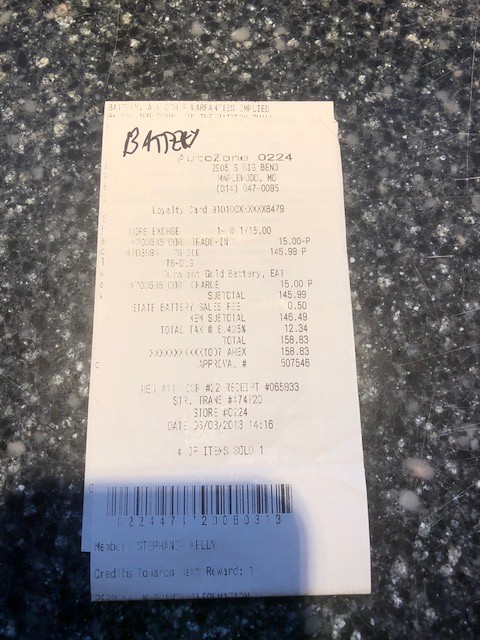This image depicts a white AutoZone receipt centered on a black granite countertop. The receipt, which is rectangular and covered in black text, has "battery" handwritten in black ink at the top left corner, indicating it's likely for a car battery purchase. Detailed information includes the AutoZone store number 0224, the store's address and phone number, loyalty card details, and various items with their prices. A barcode is located near the bottom of the receipt. The total purchase amount is $158.83, paid with an American Express card. A shadow in the bottom left corner suggests the photo was taken with a phone, reflecting the device on the countertop.